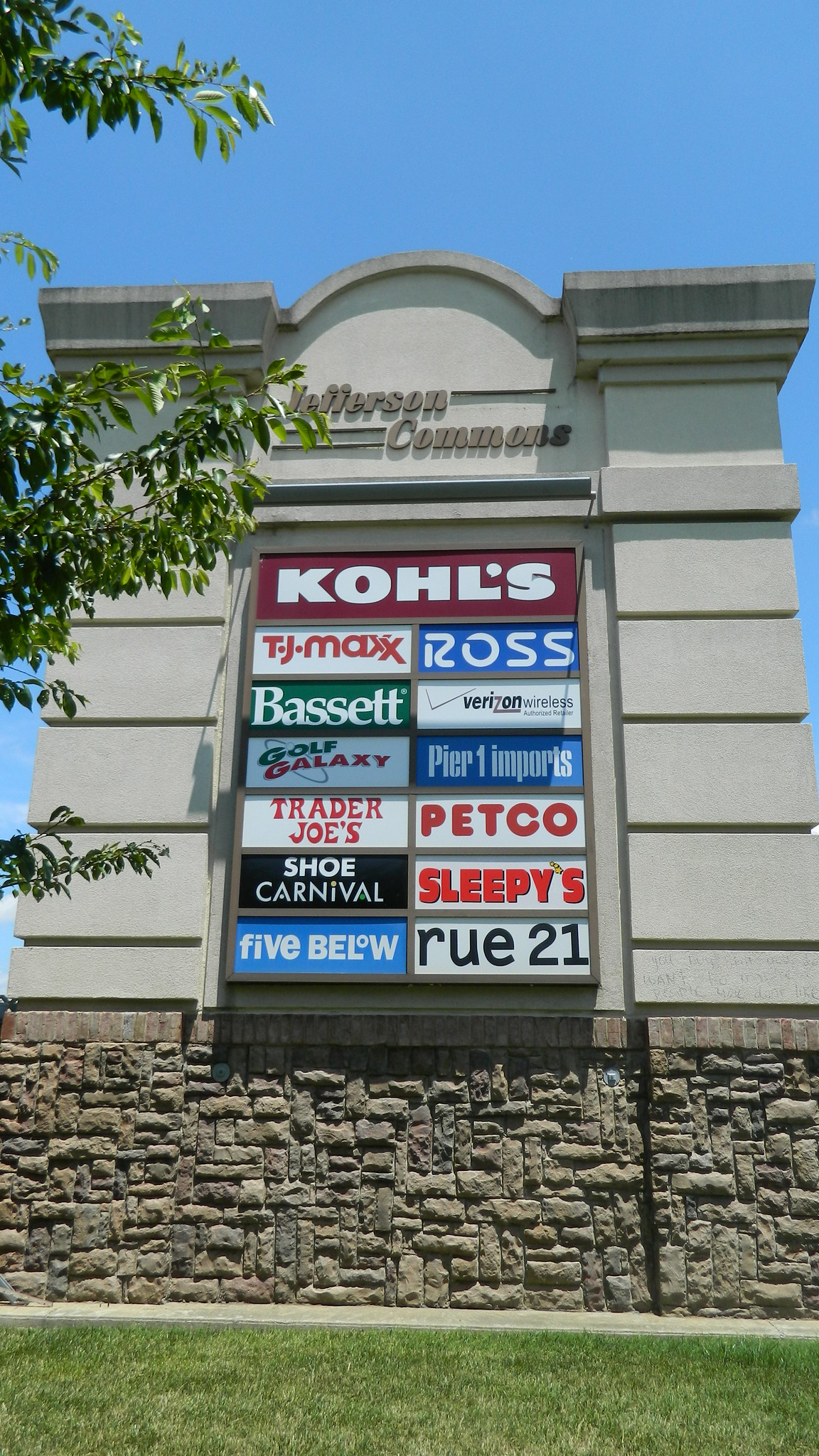The photograph showcases an imposing entrance sign for Jefferson Commons, a shopping plaza, during daylight hours. The sign, crafted from cement and concrete with a taupe body and arched top, prominently features the plaza's name "Jefferson Commons" at the top in cursive writing. Below the main title, the sign displays a list of stores, each on a colored background. At the top, "Kohl's" is shown in white text against a burgundy background. Below Kohl's to the left, "TJ Maxx" in red letters, followed by "Bassett," "Golf Galaxy," "Trader Joe's," "Shoe Carnival," "Five Below," and "Rue 21." On the right side, beneath Kohl's, is "Ross" with blue background and white text, followed by "Verizon Wireless," "Pier 1 Imports," "Petco," and "Sleepy's." The base of the sign is framed by a stone wall, leading to a neatly maintained patch of green grass in the front.